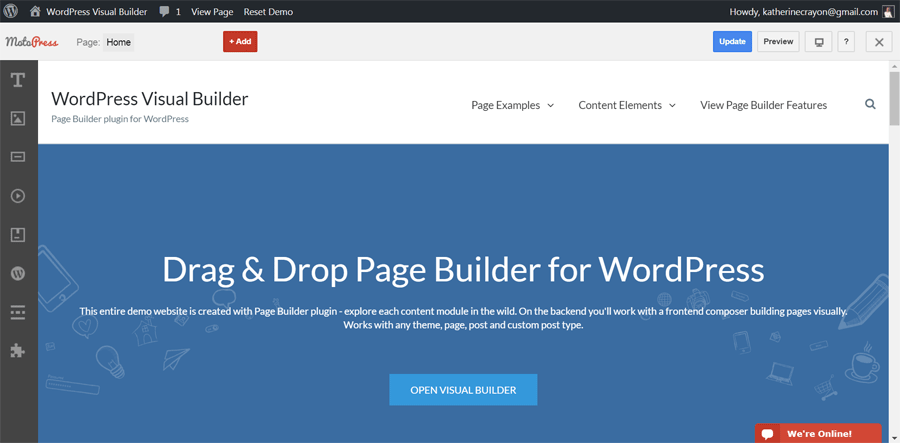**Detailed Caption:**

The image is a screenshot of a website designed for building blogs, displaying an interface that suggests familiarity with WordPress. At the top, a black navigation bar is visible, containing various tabs such as the WordPress icon, WordPress Visual Builder, one message notification, View Page, and Reset Demo. To the right of this bar, the user is greeted with "Howdy, Catherine Rayon" followed by an email address, "catherinecrayon@gmail.com," and an icon that appears to represent a person.

Below this, a grey band indicates "Malta Breeze - Page Home" with buttons labeled "Red Ad Box" to the right, followed by "Update," "Preview," a computer screen icon, and a close box icon. Down the left-hand side, there's a dark grey column with light grey symbols representing various functionalities: a "T" for text, an image icon, a rectangular shape with a line, a play button, a round play icon, a save icon, a WordPress logo, a hamburger menu (with potentially zigzaggy middle lines or three dots), and at the bottom, a puzzle piece icon.

Further down, there is another horizontal navigation bar, this one white with black text that reads: “WordPress Visual Builder, Page Builder Plugin for WordPress, Page Examples, Content Elements, View Page Builder Features” accompanied by a search icon. A vertical scroll bar is present on the right-hand side.

In the main content area, there's a blue background decorated with cartoon images of a light bulb, phone, tablet, quotation mark, paper plane, coffee cup, pen, and pencil. Overlaying this background is white text that reads: "Drag and Drop Page Builder for WordPress. This entire demo website is created with page builder plugins. Explore each content module in the wild. On the back end, you will work with the front end composer, building pages visually. Works with any theme, page, post, and custom post type." 

Below this section, there's a lighter blue rectangle with the text "Open Visual Builder" in white. At the bottom of the page, a red rectangle featuring a white speech bubble contains the text "We're online."